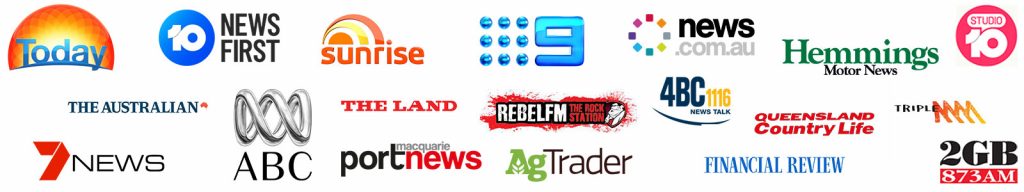A detailed screenshot of a landing page showcases an array of diverse logos from different media outlets and organizations:

1. **Sun-like Image**: At the top, there is a semi-circular sun-like icon filled with bands of gradient orange, yellow, and white semi-circles. Below the sun, "today" is written in bold blue letters with some cyan blue and a dark blue curved line underneath.

2. **"10 News First" Logo**: A dark blue circle features a white bold "10" with a 3D blue touch on the left side. Beside it, in bold black text, it reads "News First".

3. **Sunrise Logo**: This logo displays the word "Sunrise" in orange. The accompanying icon is a half-circle with orange, gold, yellow, and pinkish bands blending into dark orange edges.

4. **Channel 9 Logo**: Three equidistant cyan and dark blue circles aligned to form the number "9".

5. **Pinwheel-type Logo**: Comprising multiple squares in a circle, the colors rotate from red, pink, black, cyan, blue, teal, greenish-yellow, gray, and orange. Below it, "News" is written in bold black, followed by ".com.au" in gray, indicating its Australian domain.

6. **Hemmings Motor News**: This simple logo features "Hemmings" in bold green text and "Motor News" in bold black text.

7. **10 Studios**: A dark red pill-like shape with a small underline contains "Studio" written in red on a black and white background. It includes the number "10" with a dash around the "A" in red.

8. **The Australian**: Displaying dark blue text with a hash of red outside. Under it, the **7 News** logo features a red, stylized number "7" followed by "News" in black.

9. **ABC Logo**: A silver and gray corkscrew or spring-like shape is turned sideways with "ABC" written underneath in bold black.

10. **The Land**: Written in bold red, "The Land" is straightforward. Below it, "Macquarie Port News" is featured in bold black for "Macquarie" and bold red for "News".

11. **REBEL FM Logo**: Exhibiting a blood-splatter-like design, "REBEL FM" is written in white with a black border to the right of "The Land".

12. **The Rock Station**: This features a dark black tank-like image with "the rock station" written underneath in red.

13. **A&G Trader**: Next to "Macquarie Port News", the logo displays a stylized "A" with a white plant growing through it and a lowercase "g". "Trader" is written in black.

14. **4BC News Talk**: This logo shows "4BC" in dark blue and "news talk" underneath in the same color, followed by the yellow frequency "1116" with a dark blue band underneath.

15. **Financial Review**: Bold blue text spelling "Financial Review".

16. **Queensland Country Life**: Above "Financial Review", this text is in bold red.

17. **Triple M**: "Triple" is written in bold black, followed by two M’s in gradient orange and yellow.

18. **2GB 873 AM**: "2GB" is in bold black with a red rectangle below, and "873 AM" written in white within the rectangle.

The overall page features a white background, lending clarity and distinction to the variety of logos displayed.